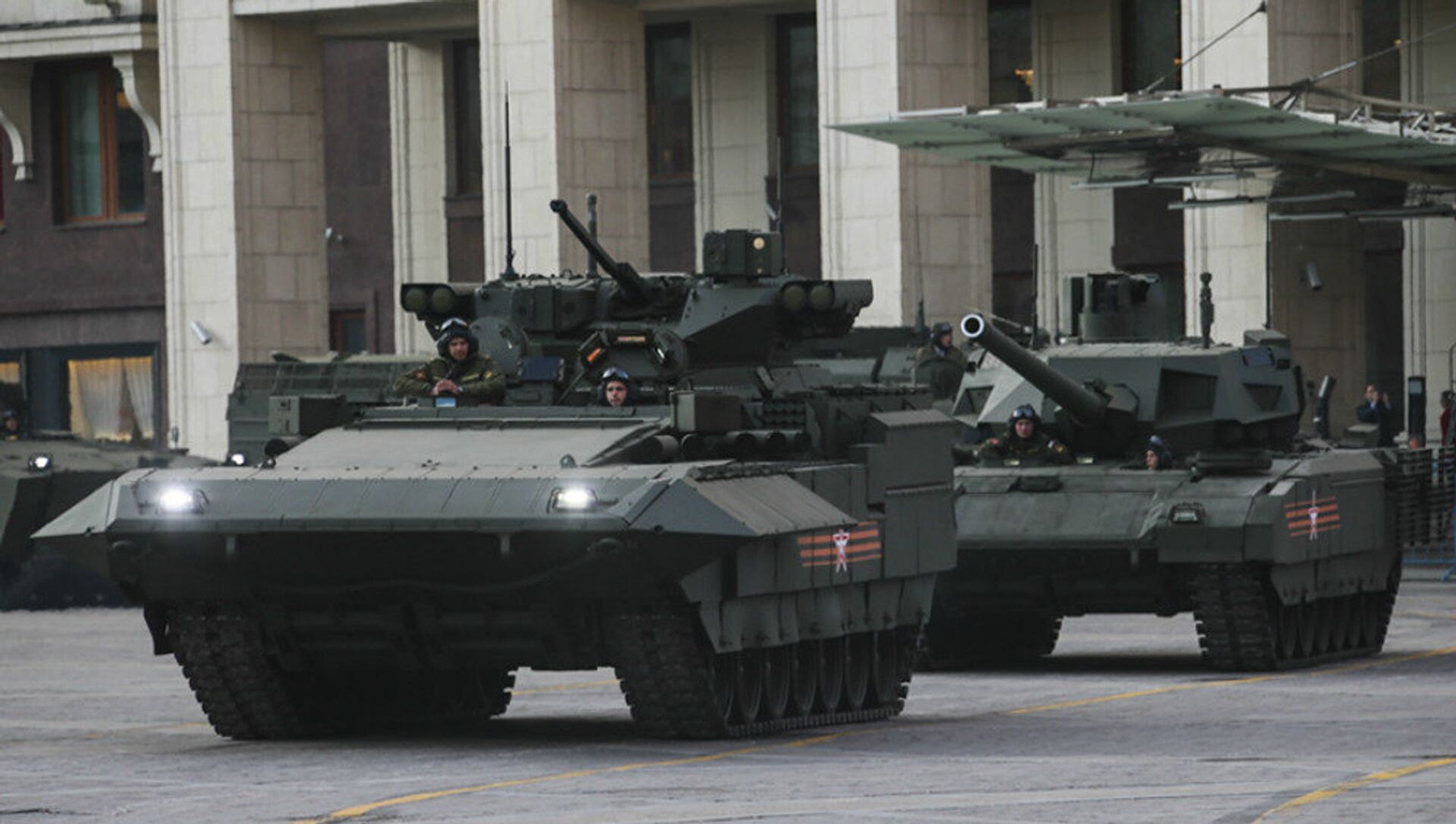The image captures a detailed outdoor scene featuring two distinct military armored vehicles positioned in what appears to be a city street lined with large buildings or apartment complexes. The front vehicle is an armored tracked vehicle equipped with a small turret-mounted cannon flanked by rocket pods. Its white LED headlights are illuminated, and it bears a distinctive insignia of three orange stripes over a white star on its side. Two soldiers are visible, turned out at the front of this vehicle.

Behind it, a lower-profile tracked tank mirrors the insignia of three orange stripes over a white star. This tank boasts a longer cannon extending over its front, with two soldiers similarly turned out. Both vehicles seem to be parked or stationed, poised as if ready to move toward the bottom left corner of the photograph. Additional military vehicles are visible in the background, evidencing a larger military presence. The backdrop features numerous windows and structural beams, likely indicating residential buildings or a densely built urban area. The photograph captures a moment of stillness amid the potential for movement and action, framed by the watchful cityscape.